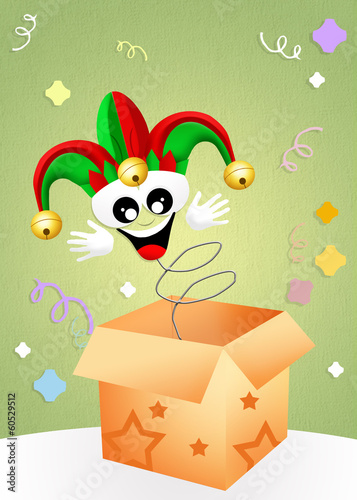This image is a digitally created stock photo with a cartoonish, card-like appearance. It is vertically aligned and showcases a playful scene centered around a jack-in-the-box. The bottom half features a brown box adorned with star decorations, positioned at a diagonal angle on a white table. The box’s flaps are folded down, revealing a spring emerging from the center.

Attached to the spring is a vibrant and animated jack-in-the-box character. This character has strikingly large black and white eyes with prominent pupils, a wide-open mouth showing a red tongue and a row of top white teeth. It also has two white gloved hands extended outward. The character is wearing a whimsical green and red jester hat, adorned with jingle bells at the tips.

The background is a light green hue, accentuated with swirly lines and various floating shapes in white, light purple, and yellow. Additionally, there are confetti-like dots in colors such as yellow, white, blue, and purple. Across the entire image, a translucent watermark that reads "Adobe Stock" is visible. In the very lower left corner, vertically printed, is another "Adobe Stock" watermark followed by the number "60529512," indicating the stock photo identification.